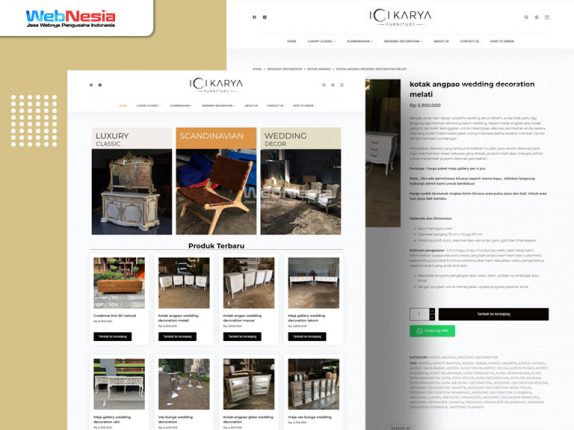The image appears to be a detailed screenshot of a catalog page from the website WebNesia, showcasing products from the Sicaria Furniture line. At the top of the page, "WebNesia" is prominently displayed, with "Web" in blue and "Nesia" in red. The left side of the screenshot features a brown banner taking up about a third of the image. The core of the screenshot is dedicated to showcasing various furniture items arranged under different categories such as "Luxury Classics," "Scandinavian," and "Wedding Decor." The Scandinavian section is highlighted in orange, while the Wedding Decor section has a stone gray or beige caption. There are around 12 different items depicted, including dressers, various types of chairs and tables, and storage units. Each item is accompanied by a brief description and a black rectangle likely representing a "Buy" or "Find Out More" button. The page also illustrates potential wedding setups, including display tables and lighting arrangements, suitable for both purchasing or renting for wedding decorations.